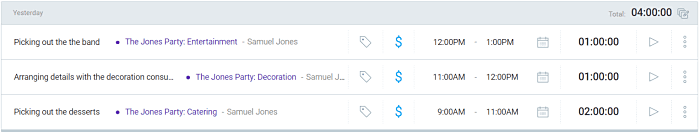This screenshot captures an organized summary of activities from the previous day, situated beneath a gray header bar. On the top left of the header, the label "yesterday" is displayed, while the top right records a "total 4 hours." 

Below the header are three detailed sections, each encapsulating distinct events coordinated by Samuel Jones for the Jones Party:

1. **Picking Out the Band**:
    - **Event**: The Jones Party Entertainment
    - **Organizer**: Samuel Jones
    - **Time**: 12 p.m. to 1 p.m.
    - **Duration**: 1 hour

2. **Arranging Details with the Decoration Consultant**:
    - **Event**: The Jones Party Decoration
    - **Organizer**: Samuel Jones
    - **Time**: 11 a.m. to 12 p.m.
    - **Duration**: 1 hour (Note: The word "Consultant" is partially cut off)

3. **Picking Out the Desserts**:
    - **Event**: The Jones Party Catering
    - **Organizer**: Samuel Jones
    - **Time**: 9 a.m. to 11 a.m.
    - **Duration**: 2 hours

Each section includes a uniform set of icons: a tag symbol, a dollar sign symbol, and a calendar symbol. On the far right of every row, a triangular play button appears, followed by a vertical trio of dots.